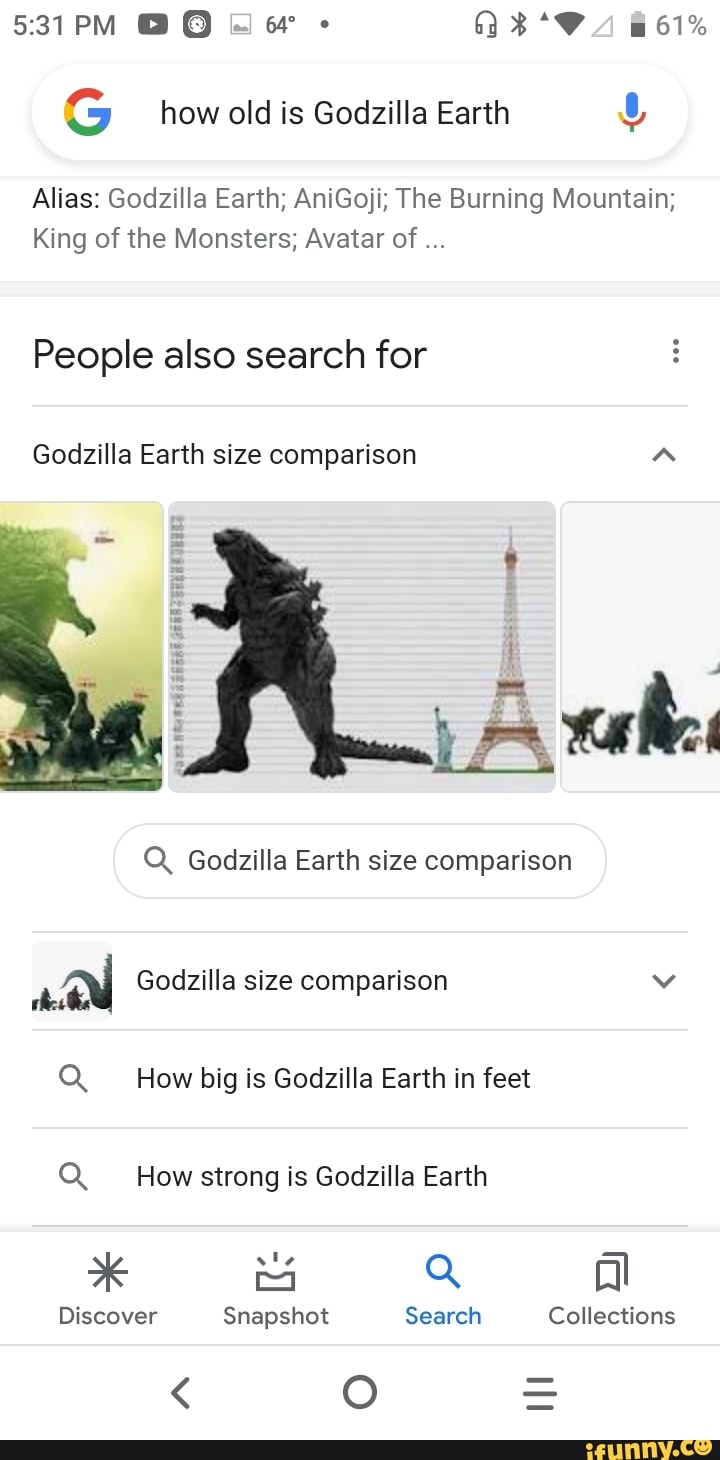A detailed screenshot of search results on a mobile device shows the query "How old is Godzilla Earth?" at the top. The time displayed is 5:31 PM and the battery level is at 61%, with headphones plugged in. The search results include multiple entries:

1. "Elias, Godzilla Earth, Inaigoji (A-N-I-G-O-J-I)" with the terms "The Burning Mountain, King of Monsters, Avatar of..." trailing off with an ellipsis.
2. Another section labeled "People also search for" features three vertical dots for additional menu options, and several related entries like "Godzilla Earth comparison" followed by an image search preview with three visible pictures.

Highlighted queries in the list include:
- "Godzilla Earth size comparison" (with a magnifying glass icon)
- "How big is Godzilla Earth in feet" (with a magnifying glass icon)
- "How strong is Godzilla Earth?"

The bottom of the screenshot displays different tabs labeled "Discover," "Snapshot," "Search," and "Collections," with the "Search" tab (represented by a blue magnifying glass icon) currently selected.